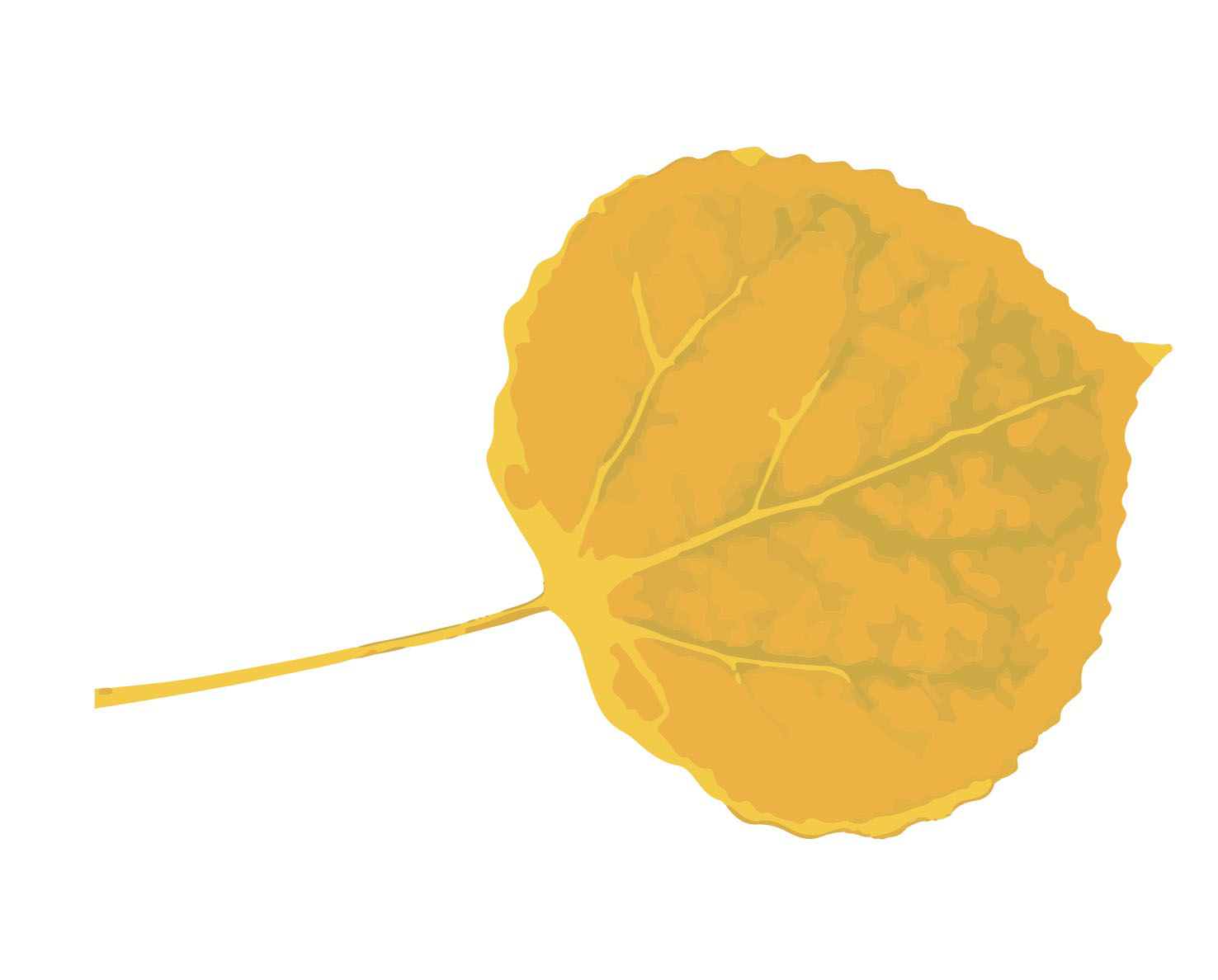The image depicts a single, illustrated leaf set against a clean white background. The leaf is predominantly mustard yellow with intricate veins that are highlighted in a brighter, cleaner yellow. There are subtle hints of light green and bluish-green that create a watercolor effect, giving the leaf varied coloring and depth. This teardrop-shaped leaf, broad and round with a pointed tip, appears to be lying sideways with its short, gold stem extending to the left. The leaf showcases a range of autumnal shades, from dark brownish-yellow to lighter mustard hues, making it reminiscent of a leaf one might find fallen off a tree during the fall season.